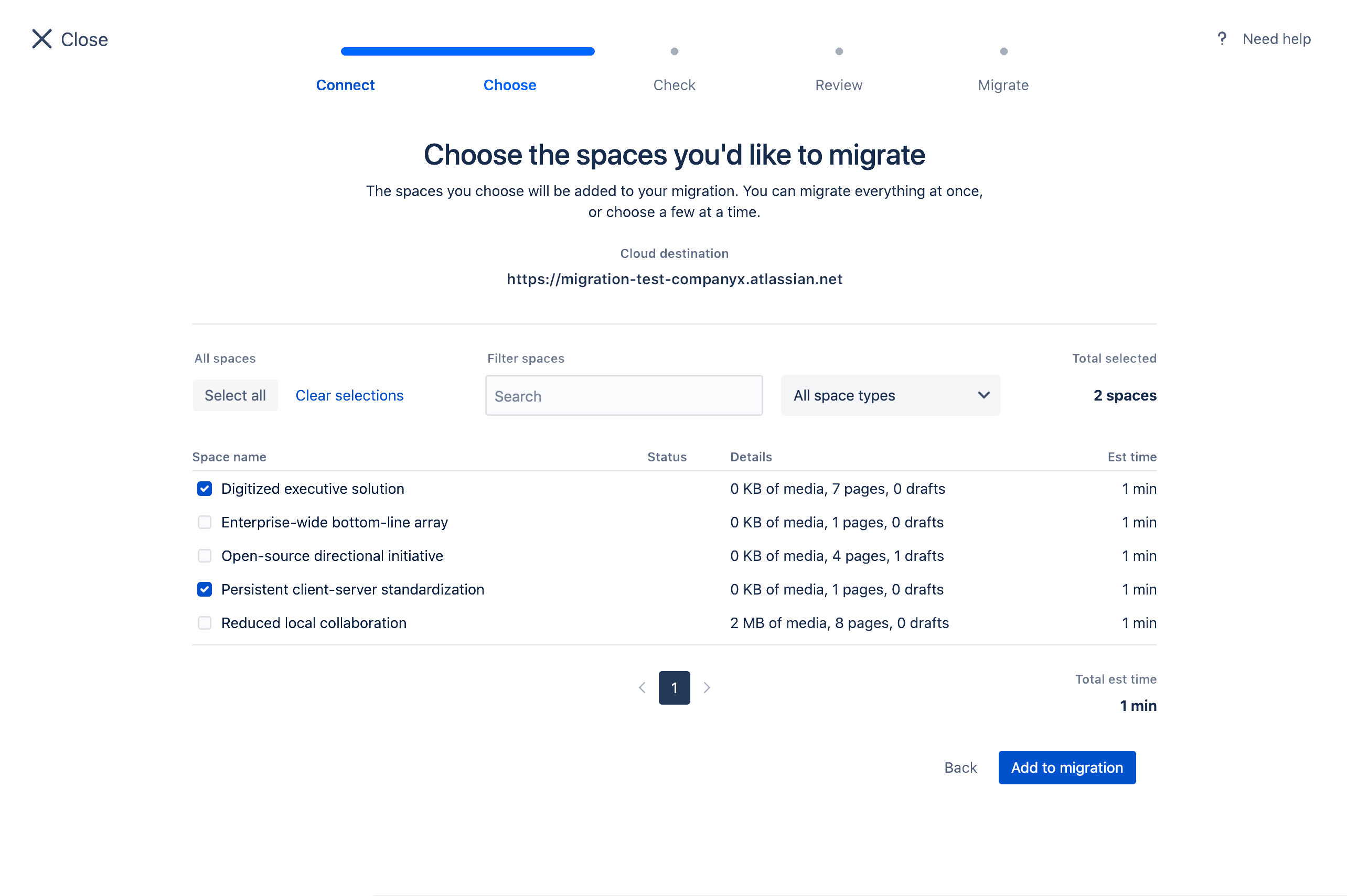A screenshot of a website interface for migrating data to a cloud destination is displayed. The web page prompts users to "Choose the places you'd like to migrate," indicating that selected spaces will be included in the migration process. Users have the option to migrate all data at once or select specific items incrementally. The website appears to be hosted on Atlassian.net, with the URL suggesting a test environment for migration efforts.

At the top, there is a "Close" button located in the upper left-hand corner. Below it, a progress bar in blue displays the current step, "Choose," within a multi-step process that includes "Connect," "Check," "Review," and "Migrate." In the upper right corner, a "Need Help?" link marked with a question mark offers assistance to users.

The main section of the page features a box with options to "Select All" or "Clear Selections," highlighted in blue. A search bar and a drop-down menu labeled "All Space Types" provide filtering capabilities. A summary shows that two spaces have been selected. Below this summary, a table lists the selected spaces, showing the names of the spaces along with their details, which include media, pages, and drafts. Each has an estimated migration time of one minute, contributing to a total estimated time of one minute.

At the bottom of the page, users have the option to "Add to Migration" via a prominent blue button or go back using a "Back" button.